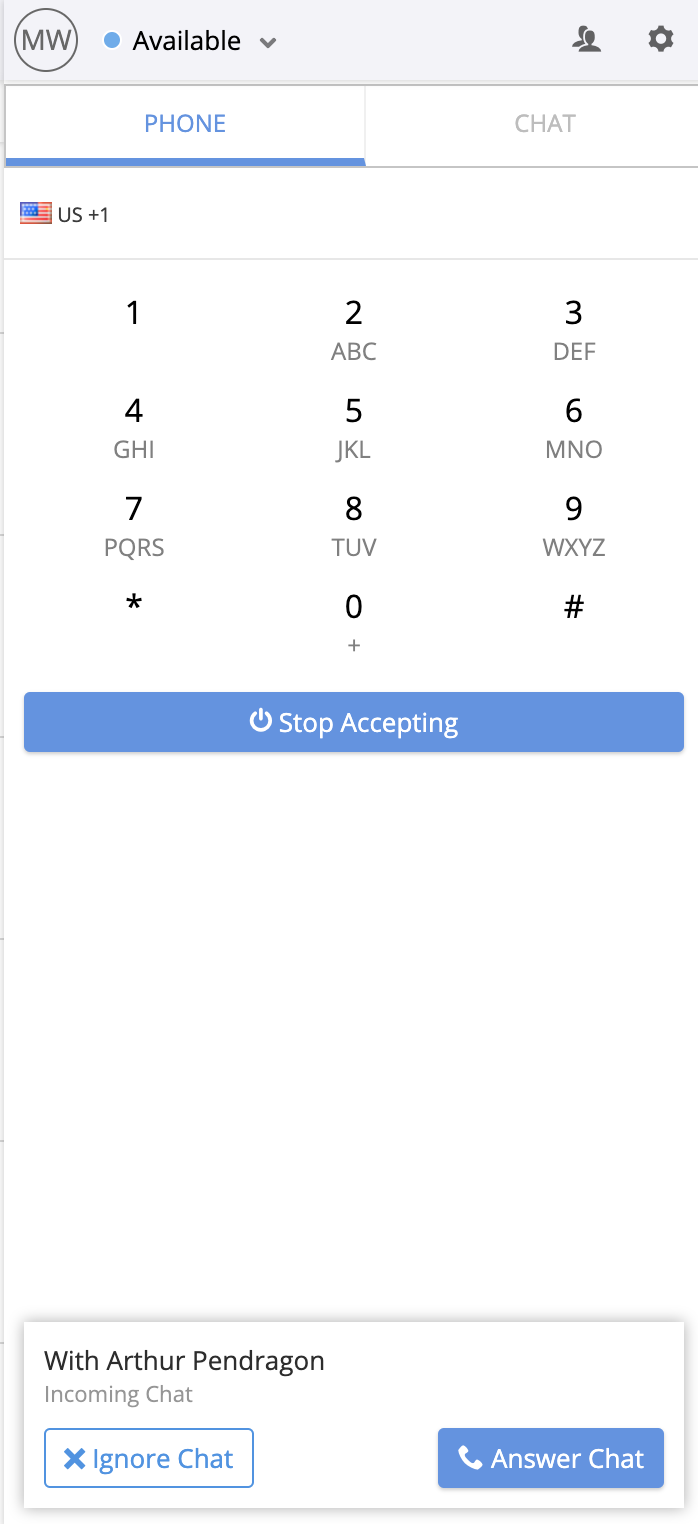In this image, we are presented with a screenshot of a phone application interface designed for making and receiving calls. The top section of the image features a grayish rectangular border. Within this border, on the top right, is a gear icon, likely indicating settings, and to its left is an icon depicting the torsos of two individuals, possibly representing contacts or social features.

On the top left corner of the interface, there is a circular icon with the letters "MW" in gray. Adjacent to this, moving to the right, is a light blue circle followed by the word "available" and a dropdown arrow, indicating the current status setting of the user. 

Below this status bar, the interface is divided into two rectangular buttons. The left button, labeled "Phone," is highlighted in blue with an underline, signifying the active tab. The right button reads "Chat." Under the "Phone" tab, we see "US +1" alongside an image of the American flag, suggesting the country code for dialing. Directly below this, the keypad for dialing phone numbers is displayed, featuring the numbers 1 through 9, an asterisk (*), zero (0), and the pound sign (#).

Further down, there is a button labeled "Stop Accepting" in white text, which likely allows the user to stop receiving calls or chats. At the very bottom of the image, a notification bar reveals an incoming chat from "Arthur and Dragon." On the bottom left of this bar, there is an option to "Ignore Chat," while on the bottom right, there is an option to "Answer Chat."